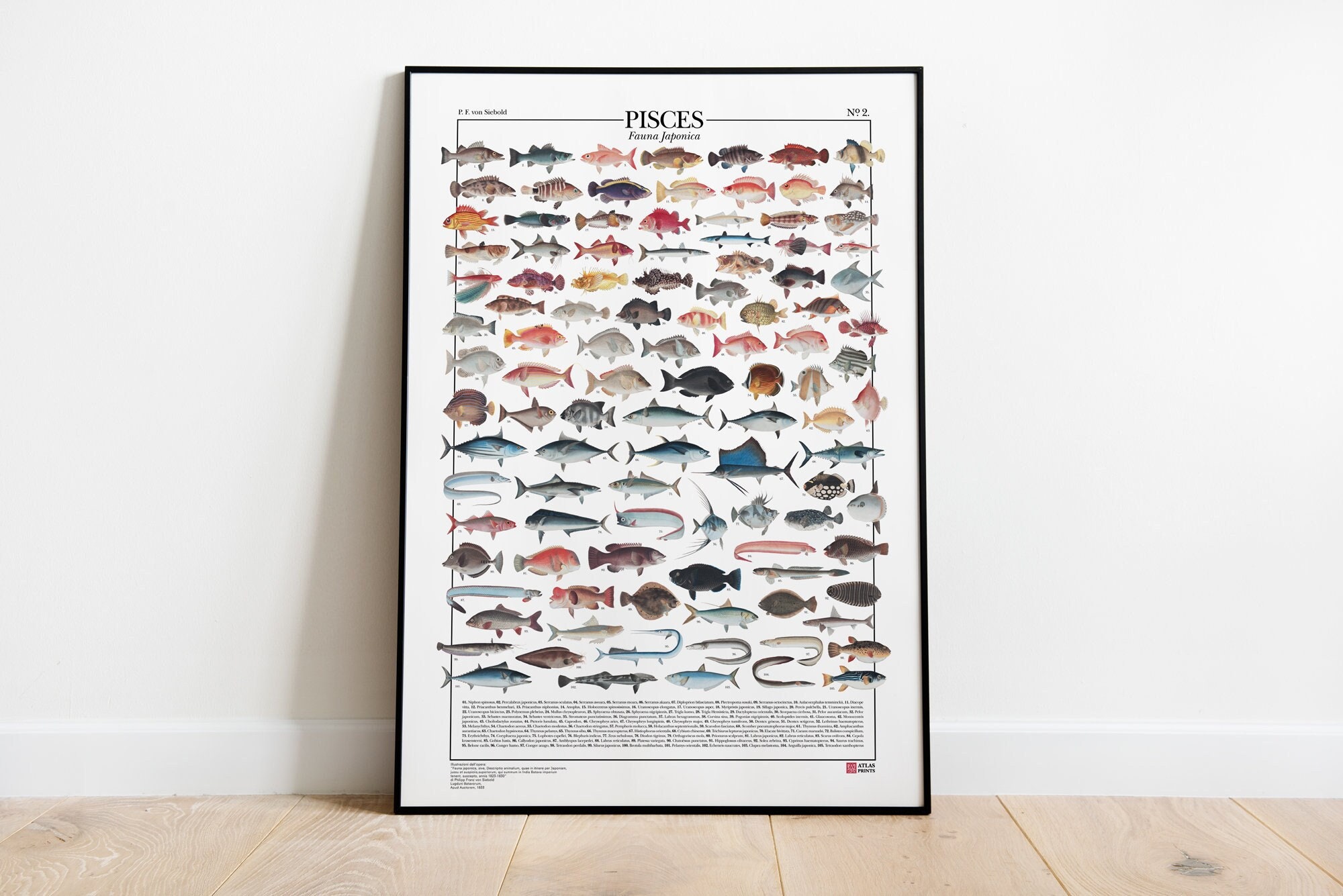This image depicts a detailed framed poster titled "Pisces," leaning against a white wall with a blonde wood floor. The black-framed poster features a plethora of fish illustrations arranged both vertically and horizontally, with each fish seemingly unique and numbering approximately between 70 to 200. The fish diversity includes species such as sharks, eels, swordfish, tuna, mackerel, sunfish, groupers, flounders, flying fish, and marlins. The vibrant illustrations showcase a variety of colors, including silver, gray, yellow, bright orange, black, and blue, against a white background. Below the illustrations is a block of fine print text that is too small to read, likely serving as a key to identify each fish. The poster, which appears to be educational in nature, is set against a baseboard, adding a subtle homey detail to the scene.